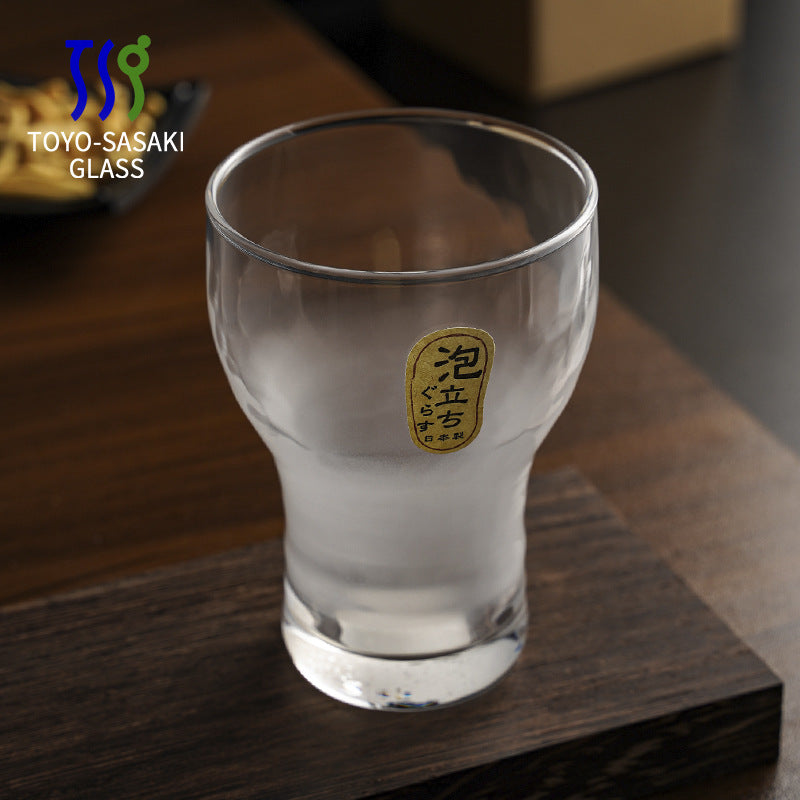The image portrays a unique glass with a clear to smoky gradient towards its base, suggesting it might be used for beverages like sake. The glass features an oblong, golden sticker adorned with Chinese or Japanese characters, adding an element of cultural elegance. The shape of the glass transitions from a wide mouth to a narrower bottom, making it easy to hold. Distinctively, there is a logo at the top left corner, composed of abstract, squiggly letters—T and S in blue and G in green—followed by “Toyo Sasaki Glass” in white font. The glass is set on a brown wooden surface, with a similarly colored or indistinct background, making it the focal point of the image.